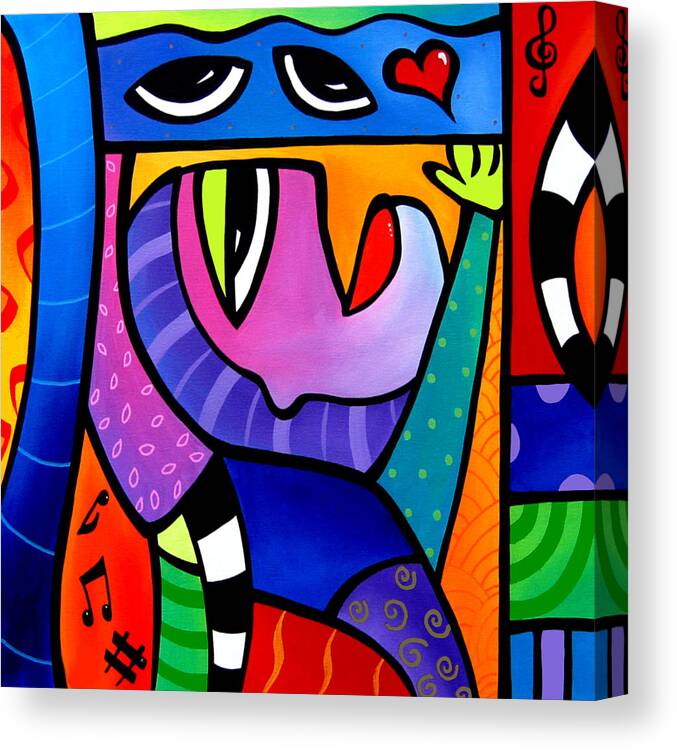The image is a vibrant, abstract canvas art piece combining various colors and elements into a captivating composition. Dominantly, it features the side profile of a face facing upwards, reminiscent of an Egyptian pharaoh, clad in a headdress. This face, painted pink, is adorned with a neon green eyelid, a stark black eye, and a white under-eye area. Above the face, on a blue background, are two oddly shaped eyes and a red heart outlined in black. The lower left corner includes musical notes, adding to the eclectic mix of motifs. The artwork is rich with a plethora of bright colors, including deep reds, oranges, purples, blues, greens, yellows, whites, and blacks. Additional elements include red and blue sections, a green arm extending upward, and various cubes in blue and purple hues. The overall composition is a vivid, highly detailed abstract piece that blends shapes, patterns, and colors into a visually stimulating experience.